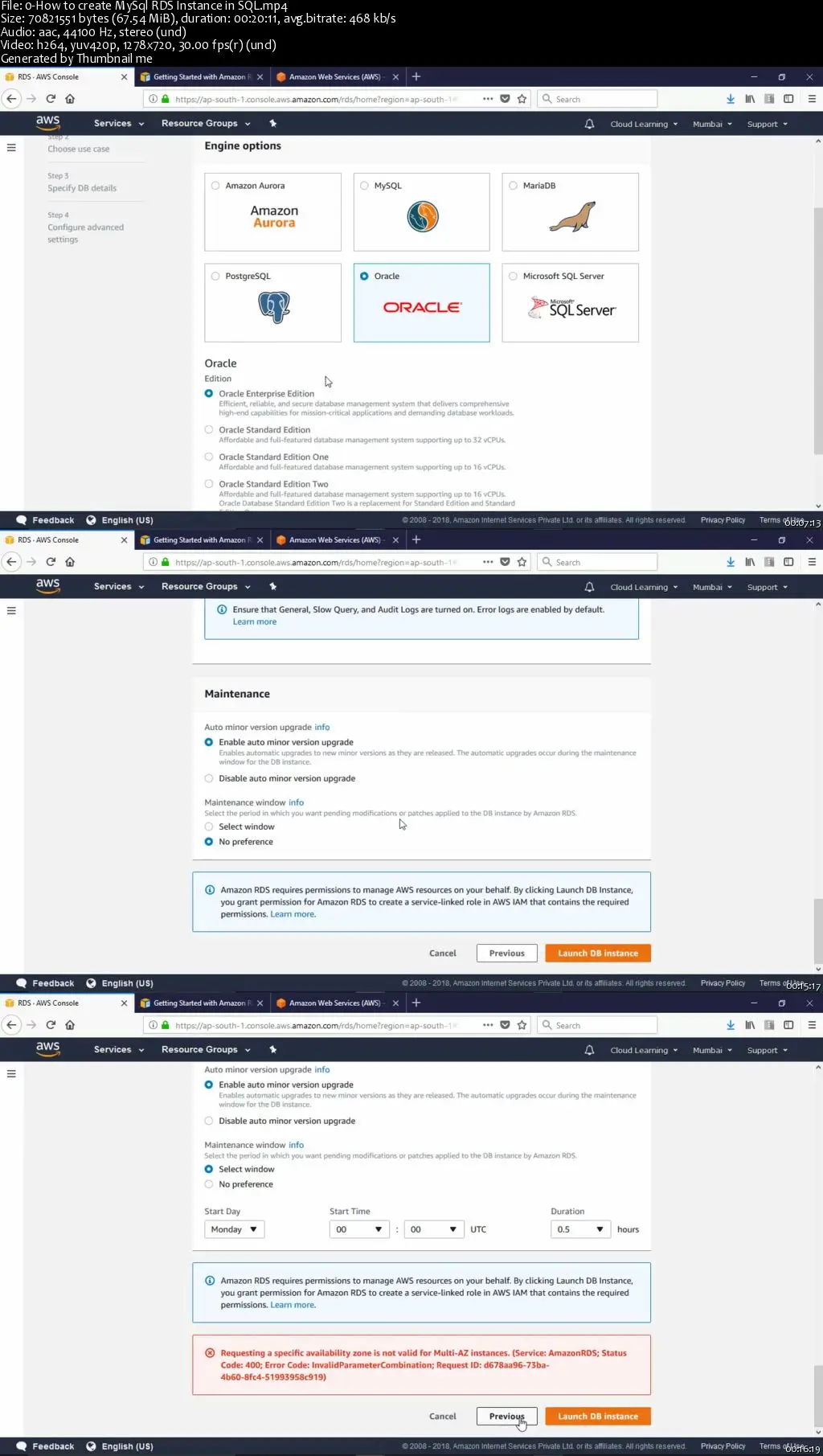The image depicts three sequential screenshots of a webpage interface, each placed one above the other, from a website related to Amazon Web Services (AWS).

The first screenshot displays the AWS Management Console for RDS (Relational Database Service). The browser tab is labeled "rds-awsconsole," alongside two non-selected tabs named "Getting Started with Amazon" and "Amazon Web Services." The main content area is divided into six selectable options, with Oracle being the selected choice. Below these options, four radio buttons allow further specification, with "Oracle Enterprise Edition" selected.

In the second screenshot, the same browser tabs are visible. The page has scrolled down to the "Maintenance" section, where the option "Enable auto minor version upgrade" is checked. The "Maintenance Window" subsection provides two choices: "Select Window" and "No Preference," with "No Preference" being selected. At the bottom of this section are buttons labeled "Cancel" (white) and "Launch DB Instance" (orange with white letters).

The third screenshot mirrors the tabs from the previous images. It also focuses on the "Maintenance Window" section similar to the second image, but this time the "Select Window" option is checked. A series of dropdown menus is visible, allowing the user to input specifics. The "Start Day" is set to Monday, "Start Time" is displayed as 00:00 UTC, and the "Duration" is set to 0.5 hours. A red alert box at the bottom of this screenshot indicates an error: "Requesting a specific availability zone is not valid for multi-AZ instances," followed by additional explanatory text in red.

This series of images illustrates various configurations and settings options within the AWS management console for an Oracle database instance.